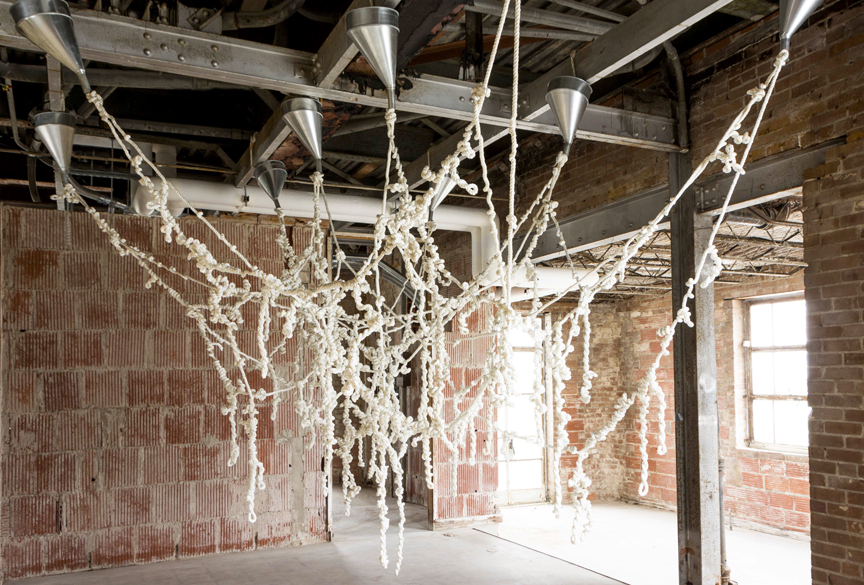This photograph depicts an intriguing art installation situated within an old brick building. The room features unevenly colored brick walls with gray grout, an light gray and slightly shiny floor, and a ceiling composed of silver metal support beams interspersed with darker gray areas. Windows along the right wall allow light to filter in, illuminating the space. Central to the installation are several large, silver, funnel-like metallic fixtures suspended from the ceiling by white ropes. These ropes are intricately tied with knots and hang downwards, almost resembling dough or a thick, stringy substance. The ropes converge to create a tangled web in the middle of the room. Additional architectural details include smaller bricks on the right wall, an arch on the top right, and metal pipes crossing the space above. Overall, the combination of these elements creates a striking visual contrast between the industrial setting and the organic nature of the installation.